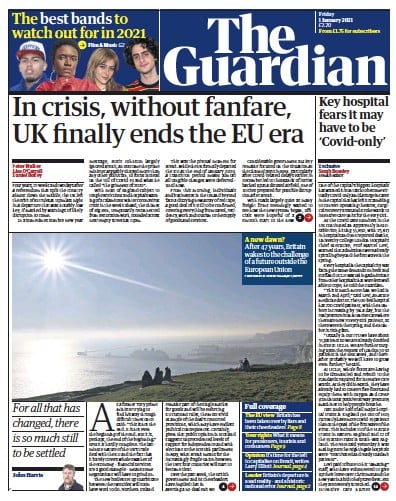The image showcases the front page of The Guardian, a prominent UK newspaper, dated January 1, 2021. Dominating the layout is a large central photograph of four individuals by the ocean, basking in the sunlight. This picture is captioned "A New Dawn," symbolizing the end of Britain's 47-year membership in the European Union, marked by the headline: "In Crisis Without Fanfare, UK Finally Ends the EU Era."

The Guardian’s banner stands out in blue with bold white lettering. Above the main image, the headline "The Best Bands to Watch Out for in 2021" hints at cultural highlights for the year ahead.

To the right of the banner, a smaller but significant headline reads: "Key Hospital Fears: It May Have to Be COVID Only," reflecting ongoing concerns about the pandemic's pressure on the healthcare system. 

At the bottom, a columnist’s quote adds a contemplative layer: "For all that has changed, there is still so much to be settled," addressing the uncertainty accompanying Britain's departure from the EU.

The front page encapsulates the pivotal moment in UK history with Brexit, set against the backdrop of the global COVID-19 crisis, while also looking forward to lighter cultural moments.